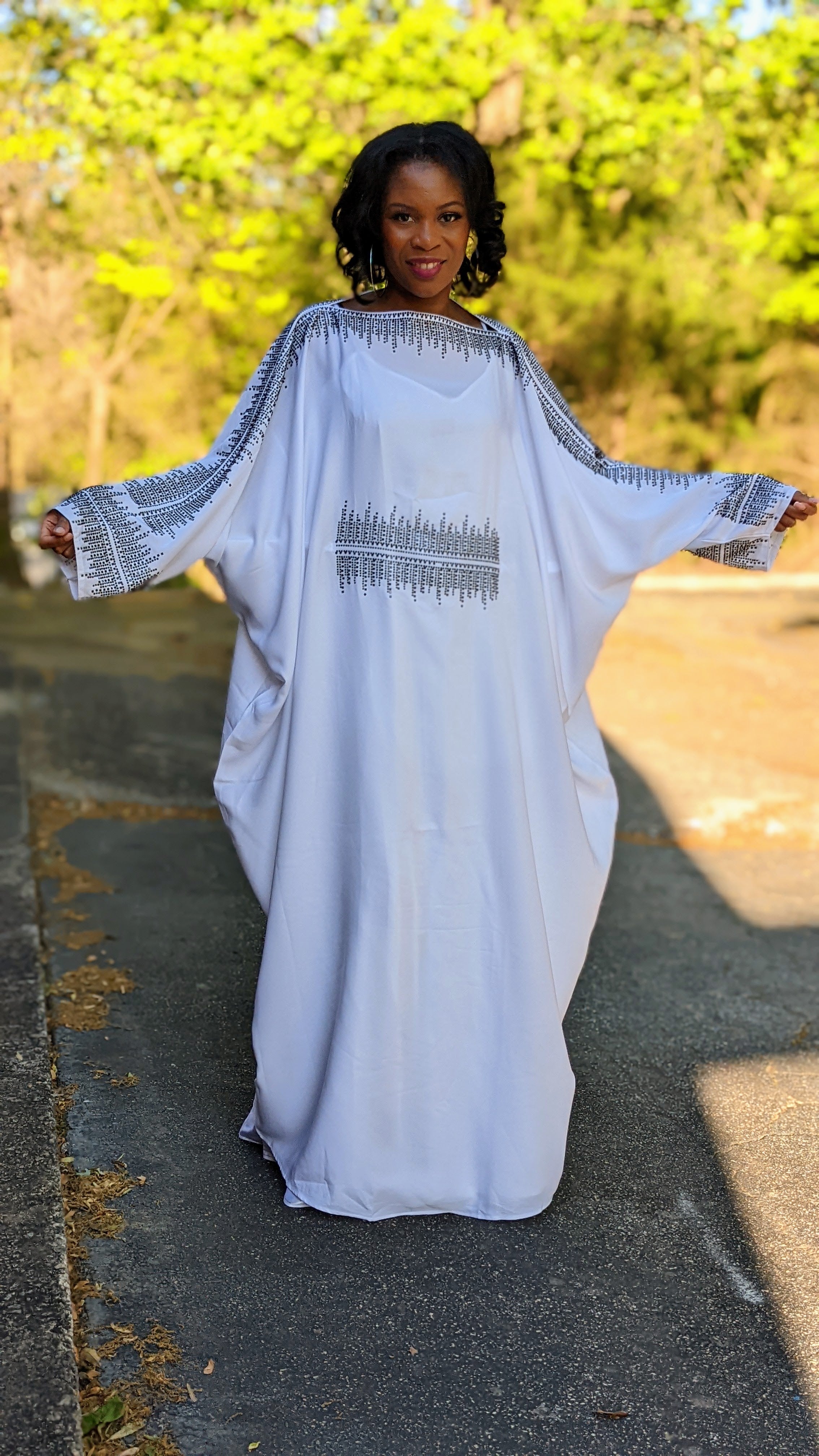The image features a young African-American woman with dark skin, brown eyes, and black, shoulder-length curly hair. She is smiling warmly, her teeth visible, with her hands outstretched to her sides. She is wearing a long, white robe that covers her entire body down to her feet, obscuring her footwear. The robe has distinct black grid-like patterns around the wrists, along the arms, across the neck, and around the waist. 

The woman is standing on an asphalt surface, which appears to be part of a sloping parking lot, with a crack filled with brown dirt nearby. In the background, lush green leaf trees bathed in sunlight are slightly out of focus. The woman herself is positioned in a shadow, with the sun shining from behind her, casting light on the trees and illuminating the setting.